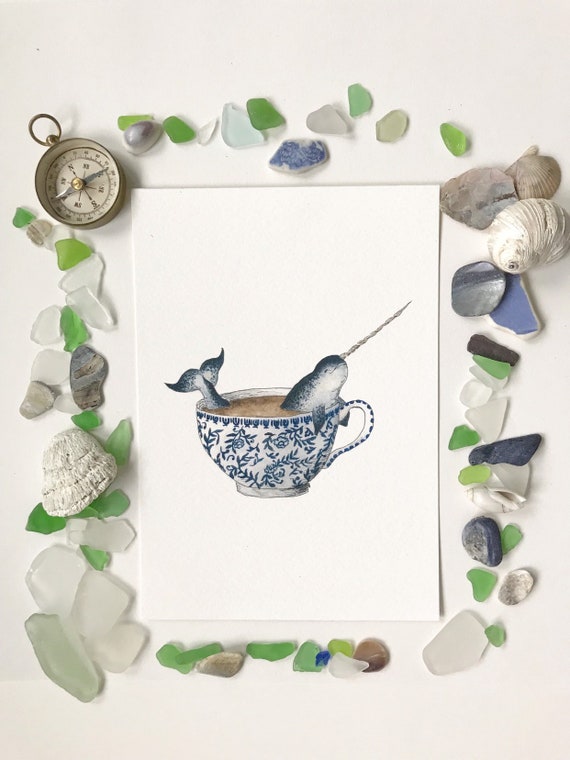This artistic image depicts a whimsical scene centered on a white and blue teacup, which contains a blue and white narwhal, complete with a prominent spike protruding from its head. The teacup is filled with a brownish liquid, potentially tea with cream or coffee. The cup itself features intricate dark blue decorations around its exterior and handle.

The main motif sits on what appears to be a piece of white cardboard, slightly lifted to cast a subtle shadow, adding depth to the image. Surrounding this central element is a creatively arranged border of various objects: white, green, and blue stones; pieces of blue and white broken pottery; sea glass; and seashells. Additionally, a compass with a ring at its top is positioned in the upper left corner.

The entire composition evokes a nautical theme, blending elements of the sea with the playful inclusion of the narwhal in the teacup, creating a charming and surreal visual narrative.